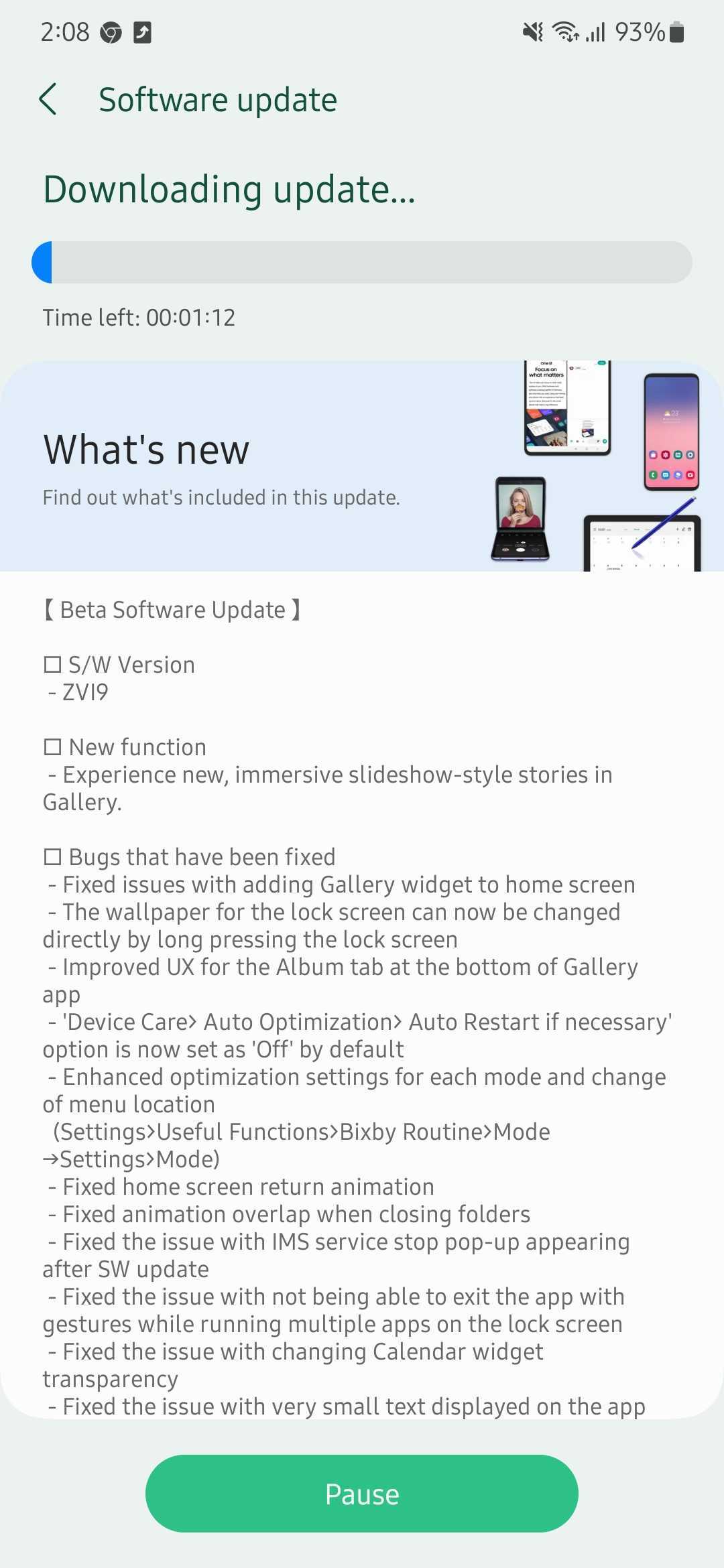The image is a screenshot of a smartphone displaying a software update notification. At the top of the screen, the time is shown as 2:08, along with the standard phone icons, including the Chrome browser logo, an upward arrow, a muted microphone, Wi-Fi signal strength bars, and a battery indicator showing 93% charge. Below these icons is a notification banner with green text and an arrow pointing left that reads "Software update - Download and install." 

A progress bar beneath this text shows the update is about 3% complete, with an estimated time remaining of 00:01:12. A blue "New" tag highlights the update details. The update is titled "Beta Software Update" and includes several detailed notes listed below:

1. **Version**: S/W Version B19.
2. **New Function**: Experience new immersive slideshow-style stories in the gallery.
3. **Bugs Fixed**:
    - Issue with adding the gallery widget to the home screen.
    - Wallpaper for the lock screen can now be changed directly by pressing the lock screen.
    - Improved UX for the album tab at the bottom of the gallery.
4. **Device Care**:
    - Auto optimization and auto restart necessary option is now set as off by default.
    - Enhanced optimization settings for each mode and change of menu locations (Settings > Useful Functions > Bixby Routine Modes > Settings > Mode).
    - Fixed home screen return animation glitch.
    - Fixed animation overlap when closing folders.
    - Resolved IMS service stop pop-up appearing after the SWB update.
    - Fixed issue with not being able to exit apps with gestures while running multiple apps on the lock screen.
    - Adjusted calendar widget's transparency setting.
    - Fixed very small text displayed on app icons.

The image also features a green "Pause" button at the bottom, which allows the user to pause the update.